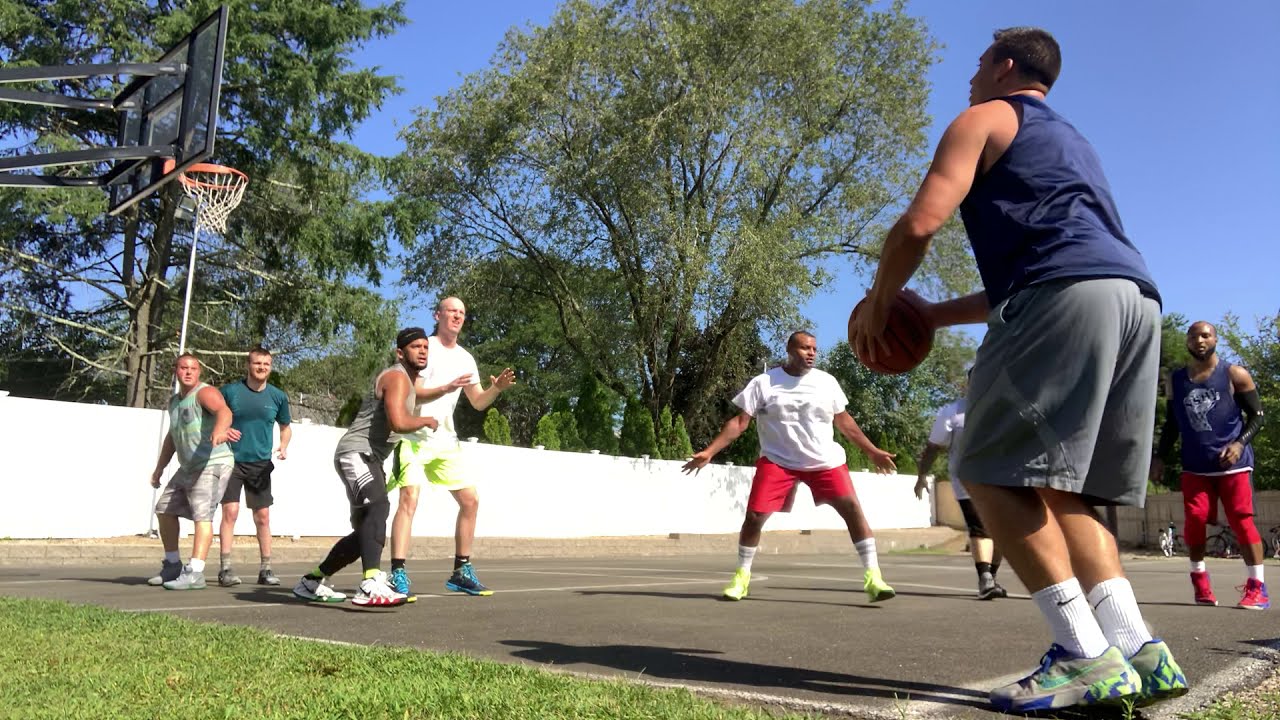In this vibrant outdoor scene set on a street basketball court reminiscent of a public park, a group of eight men are engrossed in a lively game of basketball under a brilliantly clear, cloudless blue sky. The focus is on a man to the right, poised to make a shot, holding a basketball waist-high with knees slightly bent, aiming for the hoop situated at the top left corner of the image. He is dressed in a shiny dark blue tank top, loose-fitting knee-length shorts, gray shoes with blue and green detailing, and white Nike socks. Surrounding him are other players, both black and white men, in a variety of summer clothes — some in white shirts, others in blue jerseys or teal attire — all taking defensive positions around the court. In the background, a light wooden fence lined with trees full of lush green leaves and some pine trees encloses the scene, complementing the grass that borders the court and emphasizing the picturesque, sunny day.